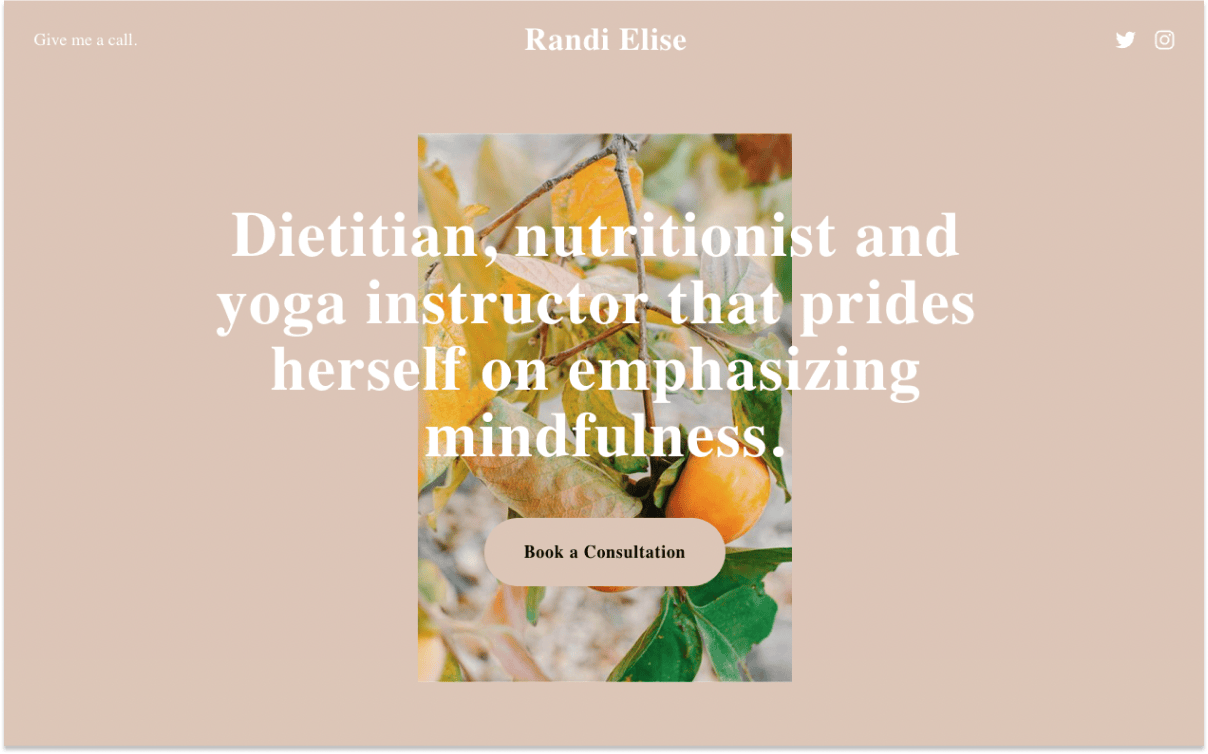This is a clean and detailed caption for the provided image description:

---

The image is a vertically-oriented mock-up of a website landing page for "Randi Elise." It features a mauve or dusty rose background. At the top left, there's a text button labeled "Give us a call." In the upper right corner, the page includes icons for Twitter and Instagram. 

Central to the design is a photograph of a fruit tree, either a peach or an apple tree, providing a natural, calming visual. Overlaying this image is large white text that spans beyond the image, proclaiming "Dietician, Nutritionist, and Yoga Instructor that prides herself on emphasizing mindfulness." 

Approximately 75% down the image, there is a button labeled "Book a Consultation" floating in the center. The bottom of the page has a subtle drop shadow, giving a slight depth effect. The rest of the page is blank, with no email links or additional information visible.

This layout appears to be a simple, clean design, possibly a template or a mock-up showcasing an option for a client.